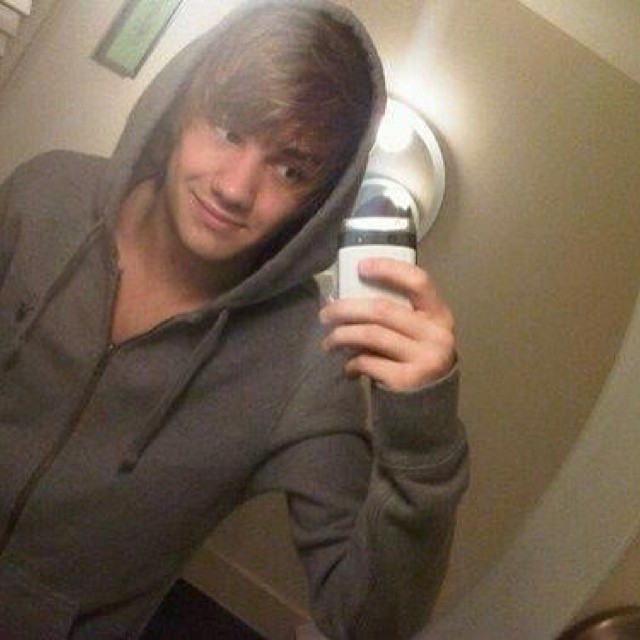The image depicts a young man standing slightly to the left, holding a white object with a rounded black top that resembles either a camera or a small container, such as deodorant. He appears to be in the act of taking a selfie. His hair is light brown, somewhat long, and falls just past his eyebrows. He's wearing a gray hoodie, which is mostly zipped up with the hood covering his head, and two strings hanging down from either side of the hood. His left hand is raised, focusing on the device in his hand while he sports a small, closed-mouth smile. The background reveals a tan wall with white trim and a shining mirror, casting a light reflection. The picture appears to be angled slightly, rotated about 30 degrees clockwise, and includes part of a metal object, possibly a doorknob or sink, in the lower right corner.